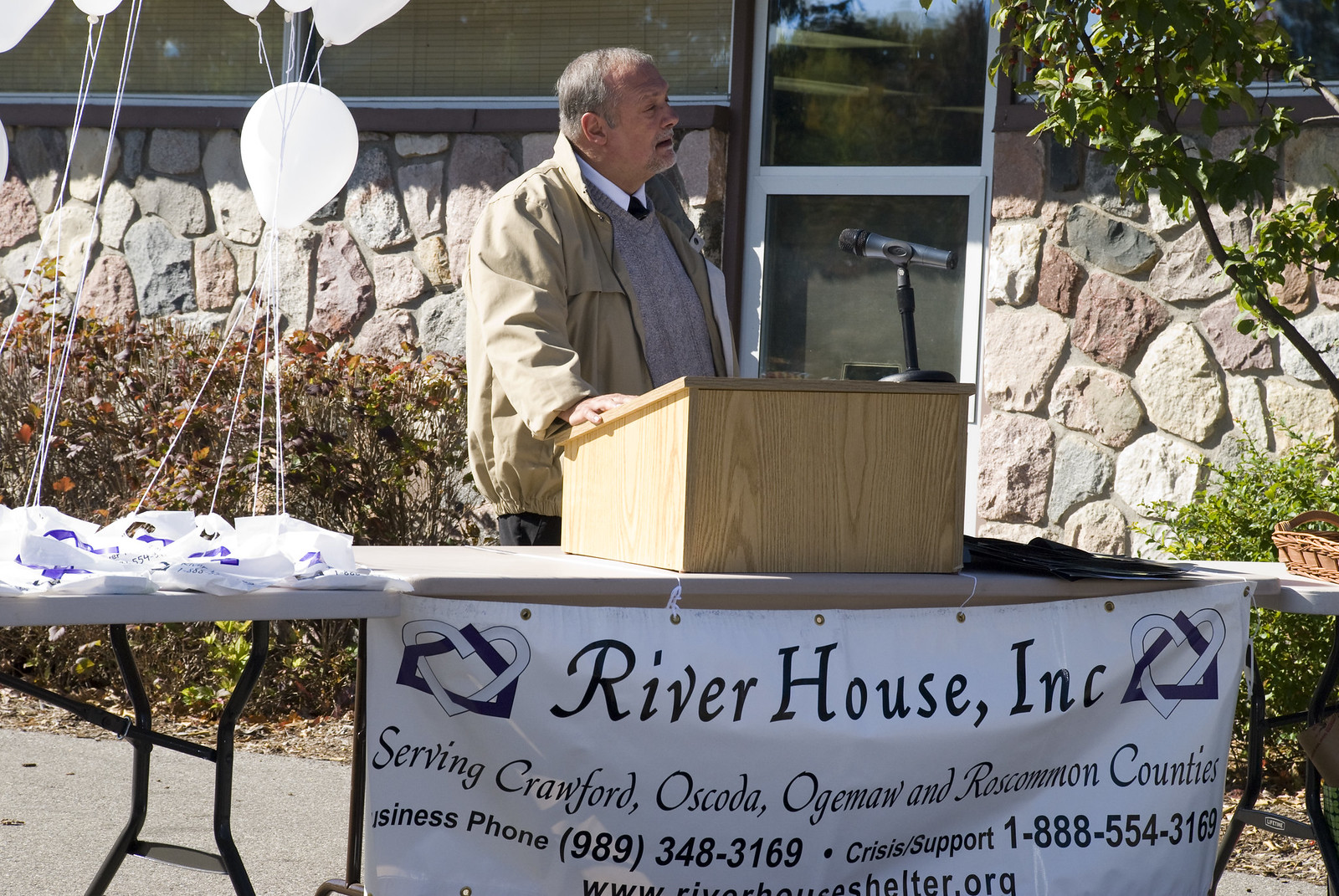An older man, likely in his 50s or 60s, is standing behind a light wood-colored podium which is placed on a standard plastic table. He has thinning white hair and is dressed in a cream-colored jacket over a white dress shirt and tie, with a gray sweater vest underneath. The man is speaking outside, in front of a building with a wall made of large, multicolored stones ranging from gray to light beige, brown, and tan. To his left, several white helium balloons float upwards, anchored by what appear to be white plastic bags with purple writing. Hanging from the table in front of the podium is a white banner that reads "Riverhouse, Inc." in bold letters, and below that, in smaller font, it states "Serving Crawford, Oscoda, Ogemaw, and Roscommon Counties" along with phone numbers for business and crisis support, as well as a website address. The surroundings include windows, a door, and some bushes, while the ground is a slightly darker shade.